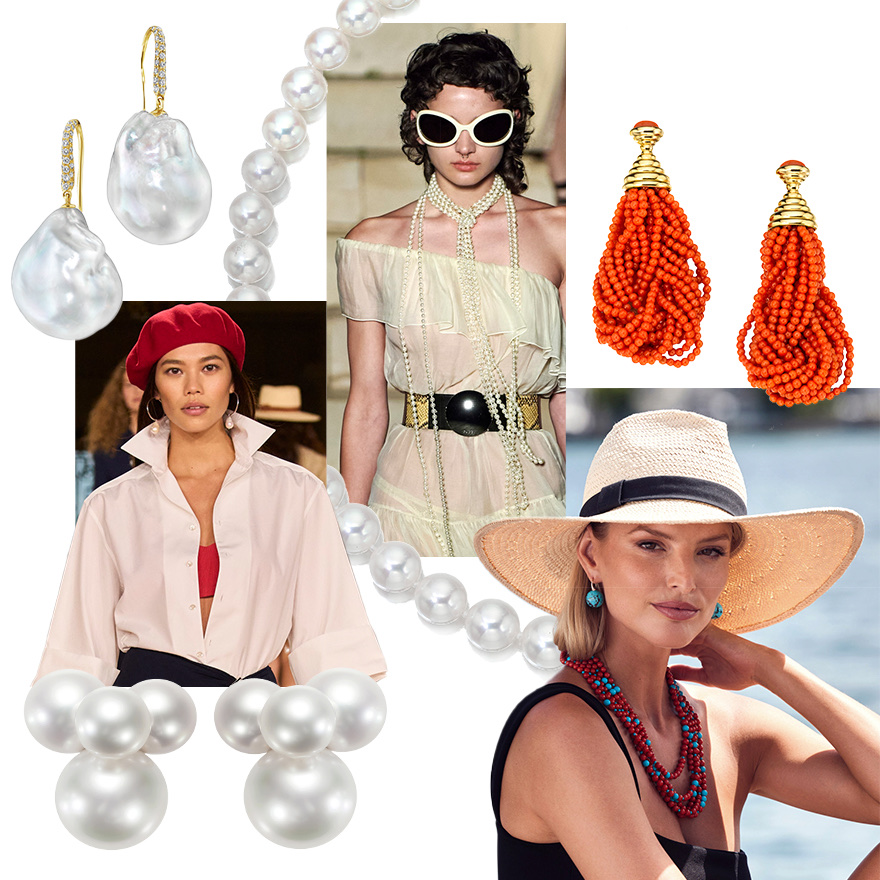The collage presents a stylish and intricate montage featuring three female models adorned in various pieces of jewelry. In the top left, a model wearing a white, long-sleeve shirt, unbuttoned except for the bottom, showcases a red bralette underneath and a red beret on her head. Behind her, two more females are faintly visible. She accessorizes with pearl earrings and an elegant pearl necklace.

In the center, another model stands out with cat-eye white sunglasses adorned with black lenses. She is draped in a see-through white lace dress, cinched at the waist with a black belt, detailed with gold accents. Her look is completed with a long strand of pearls around her neck.

The model in the bottom right, who seems to be in a beach setting, dons a wide-brimmed straw hat with a black band. She pairs her chic blue and black earrings with a striking necklace made of blue and red beads. Her outfit, a black swimsuit, complements the relaxed yet sophisticated feel of her accessories.

The jewelry pieces are prominently featured around the models: a set of misshapen, rounded pearl earrings, a traditional pearl necklace flowing from the top center to the bottom right of the collage, and an orange pair of beaded earrings with gold caps. A close-up of red bead earrings with golden tops is also displayed on the image's right side.